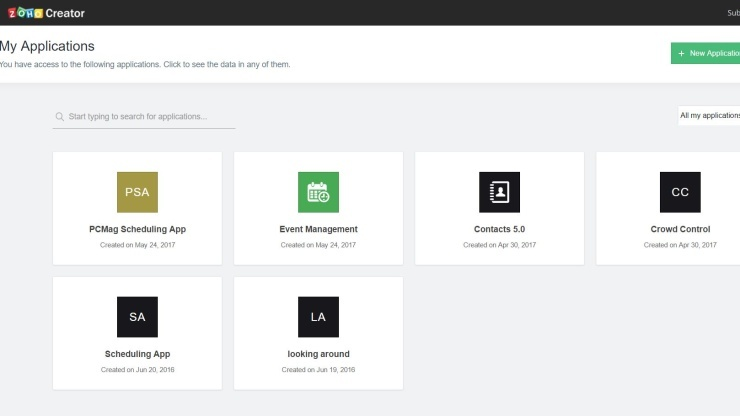This is a screenshot of an application called Zoho Creator, showcasing the "My Applications" section prominently in large black print. Below this heading, a message reads, "You have access to the following applications. Click to see the data in any of them." The interface displays six distinct applications, each encapsulated in a white box and accompanied by a uniquely colored square logo above their titles. The featured applications are named as follows: "PC Mag Scheduling App," "Event Management Contacts 5.0," "Crowd Control Scheduling App," and "Looking Around." This organized layout highlights the accessible tools and their visual identifiers within the Zoho Creator platform on the user's device.